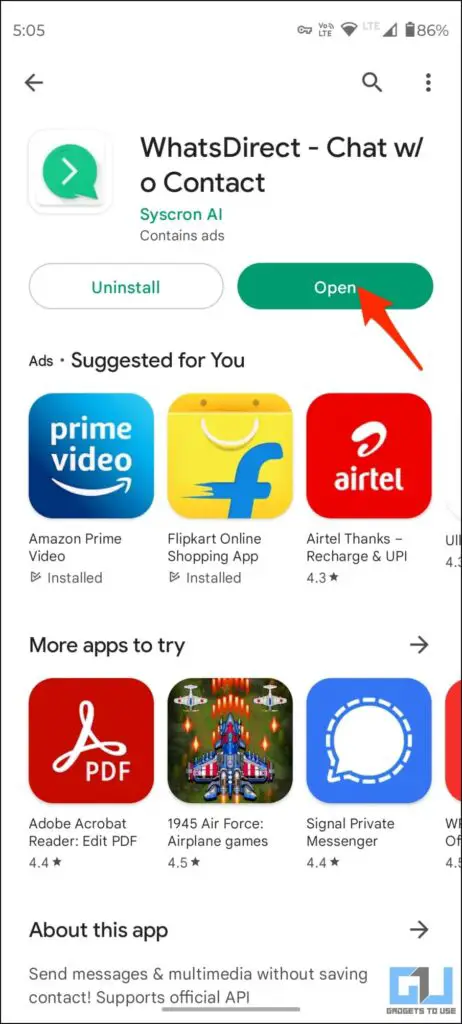The image depicts a screenshot of a smartphone application interface. The top left corner indicates the time as 5:05, alongside standard icons such as the LTE signal, Wi-Fi signal, and a battery indicator displaying 86%. The background is predominantly white, contributing to a clean and minimalist aesthetic.

At the top of the interface, there is an application named "What's Direct" with the tagline "Chat with Ocontact." This app is developed by Syscron AI and includes the notice "Contains ads." Two buttons are visible beneath the app's name: an "Uninstall" button in white with green lettering, and an "Open" button in green with white lettering. The app icon is a circle featuring a white checkmark.

Directly below, there are "Ads suggested for you" featuring various apps such as Prime Video, Flipkart Online Shopping App, and Airtel Thanks Recharging App, along with a prompt for "More apps to try." This section showcases additional recommendations like Adobe Acrobat Reader, 1945 Air Force Airplane Games, and Signal Private Messenger.

Further down, there is an "About This App" section that describes "What's Direct" as enabling users to send messages and multimedia without saving contacts, supporting the official API. In the lower right corner, a logo for "Gadgets to Use" is visible, represented by a blue and gray symbol resembling the letters 'G' and 'U'.